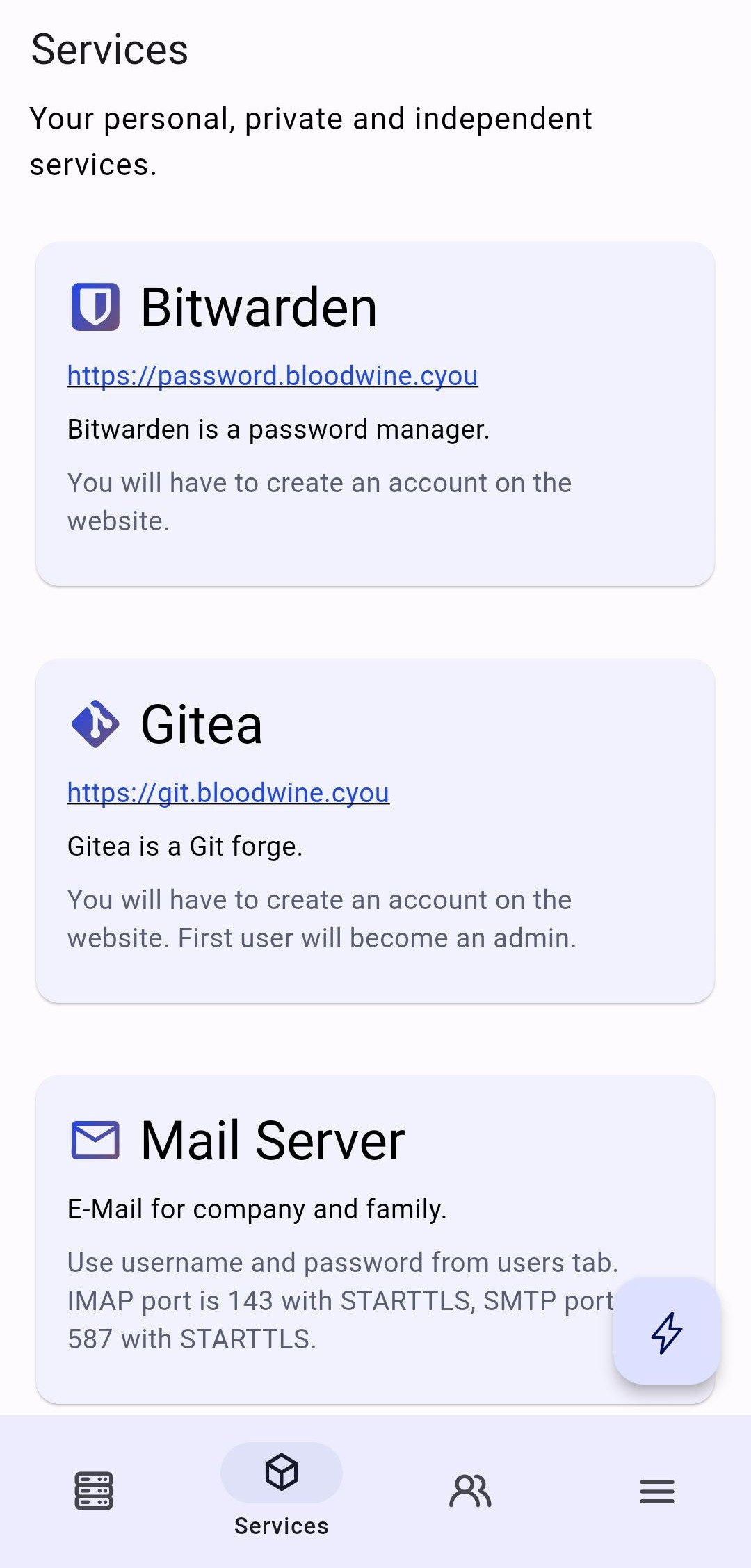This is a detailed screenshot from a smartphone showing a website. The background is predominantly white. In the top left corner, there is a large black heading that reads "Services." Beneath that, in slightly smaller black text, it says "Your personal, private, and independent services." 

Below this text, there is a blue rectangle. In the top left corner of the rectangle, there is a blue square featuring a shield icon. The left side of the shield is gray, the right side is blue with a gray border. To the right of this shield, in bold black lettering, it says "Bitwarden." Underneath "Bitwarden," a blue underlined URL reads "https://password.bloodwine.cyou." Directly below this URL, there is a black line followed by another black line separated by a small space. 

Next, there is another rectangle with a tilted blue square in the corner, which has a line extending from the top left and angling down to the bottom and off to the right. To the right of this, in large bold black text, it says "Gitea." Below this, there is another URL in blue and underlined, reading "https://gtf.org." Beneath this URL, there is explanatory text: "Gitea is for git to forge. You will have to create an account on the website first. The user will become an admin."

Following this section, there is a small space, then another item featuring an email icon in the left corner. Alongside this icon, in large bold black text, it states "Mail Server." In smaller black text below, it reads "Email for company and family." This section contains three lines of information, ending in the bottom right corner with a square that appears slightly raised but is the same color as the background. Inside this square, there is a lightning bolt icon with a dark blue border.